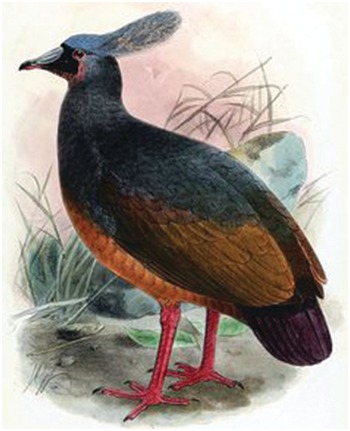This detailed hand-drawn watercolor painting depicts an uncommon bird species standing in a marshy area, surrounded by light gray-green vegetation and scattered rocks. The bird, somewhat duck-shaped, stands on muddy ground with large, distinctively pink, almost scaly feet featuring three toes in the front and a smaller balancing toe at the back, each ending in sharp claws.

The bird's body displays a striking mix of colors. Its upper part is dark gray to black, with feathers transitioning to a rich brown toward the lower wings—lighter, almost golden brown in the foreground, and darker purple tones towards the back. A light blue and cream crest decorates the top of its head, leading to its similarly colored light blue beak. The bird's head features pink cheeks and a brown eye nestled in black facial markings.

Although the background suggests an outdoor setting, it has a somewhat abstract quality, with grasses and possibly pinkish hues blending into the white backdrop. The bird faces left, perhaps on alert for prey or potential threats, adding a sense of vigilant life to the scene.